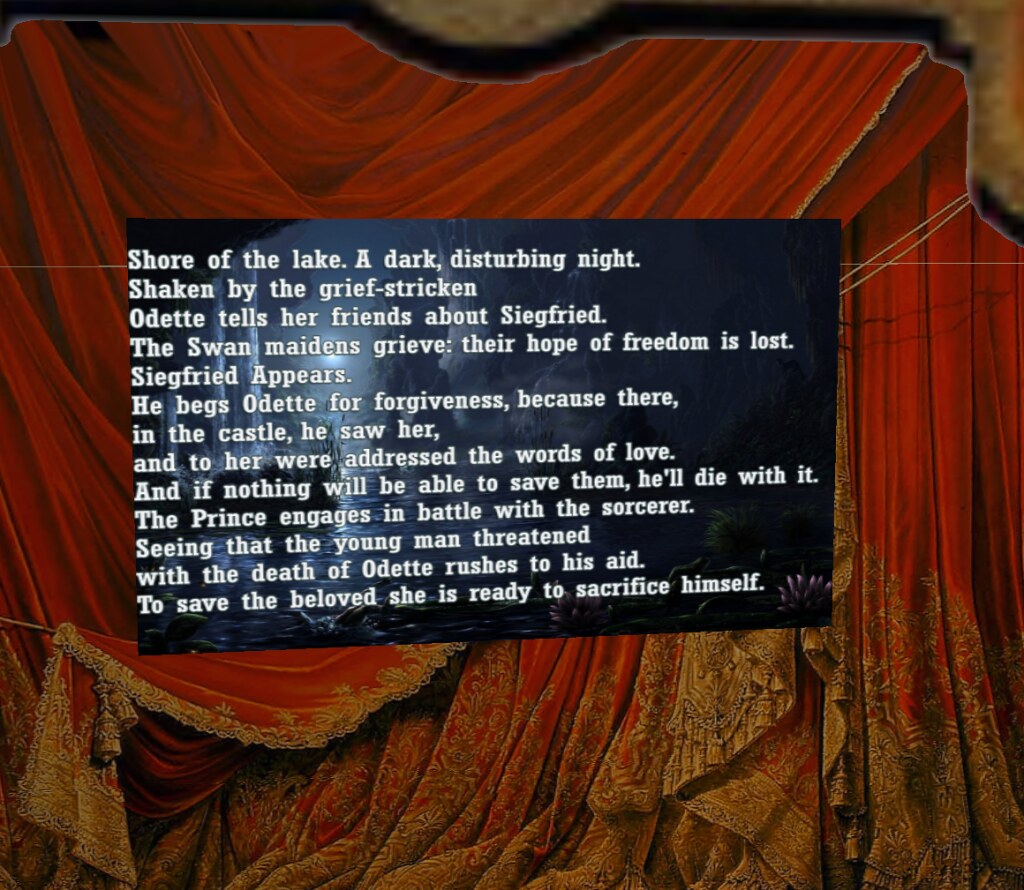In the image, white lettering overlays a dark fantasy painting of a nighttime landscape, featuring a bright star illuminating the water and white cliffs in the background. The text, set against this somber scene, reads: "Shore of the lake, a dark, disturbing night. Shaken, the grief-stricken Odette tells her friends about Siegfried. The swan maidens grieve as their hope of freedom is lost. Siegfried appears and begs Odette for forgiveness because, in the castle, he saw her and addressed his words of love to her. He vows that if nothing can save them, he will die with her. The prince engages in battle with the sorcerer. Seeing Siegfried in mortal danger, Odette rushes to his aid, ready to sacrifice herself to save her beloved." 

The poetic narrative creates an evocative and emotional scene, capturing the turmoil and passion between the characters in this dramatic moment.